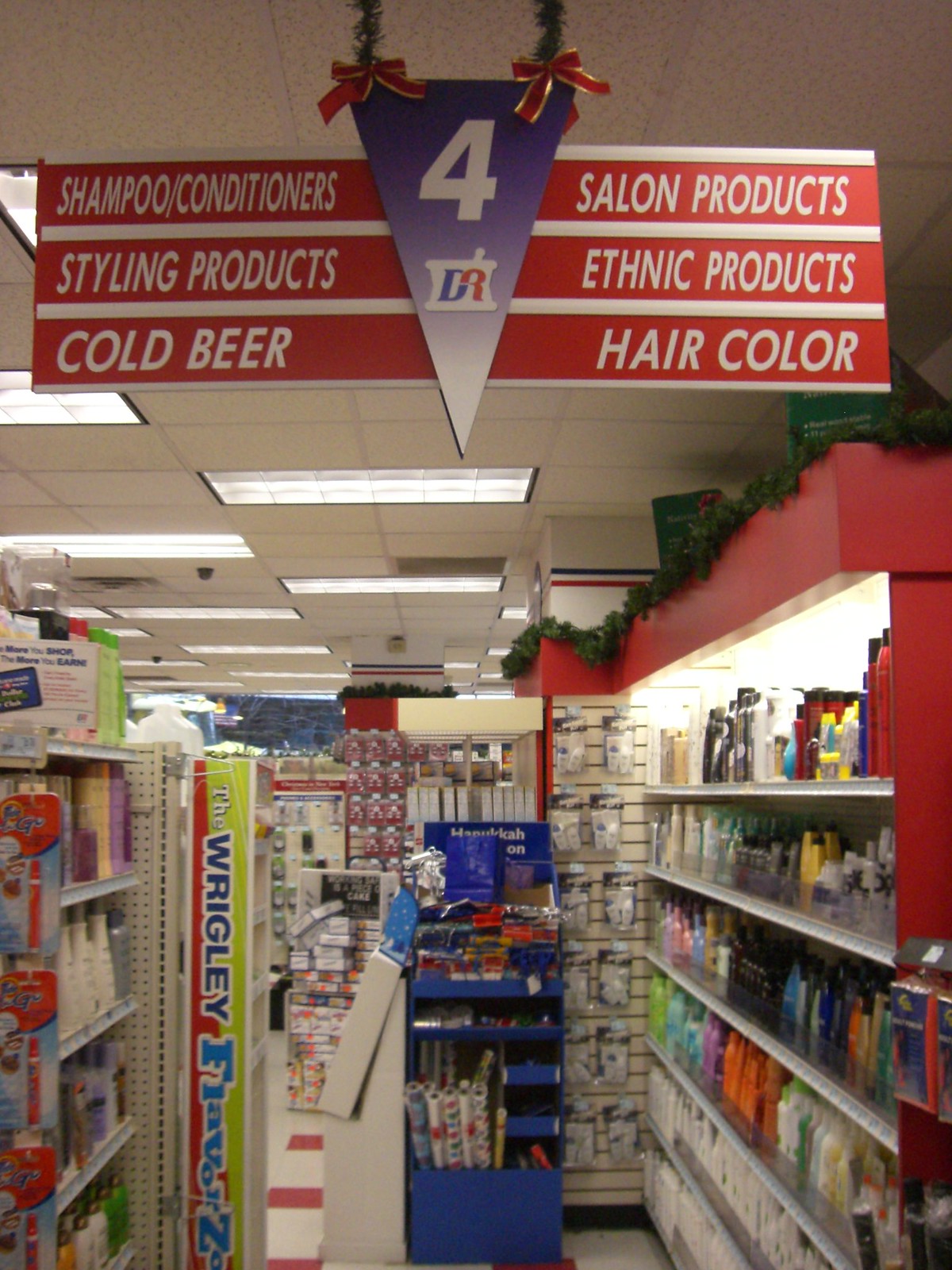This photo captures a vividly detailed scene in a drugstore aisle. Above, a red and white sign clearly lists products available in the store, such as cold beer, styling products, and shampoo on the left side, while salon and ethnic hair color products are noted on the right. A striking upside-down pyramid-shaped purple sign, displaying "4" and "DR," indicates the aisle number. 

On the left side of the aisle, a white metal shelving unit stocked with various shampoos stands out, featuring a distinctive lime-green corner at the end labeled "Wrigley" with the text oriented vertically. To the right, the wood of another shelving unit is painted red and is adorned with festive plastic decorations resembling Christmas tree foliage. Additionally, in the center of the image, a blue shelving unit adds to the organized clutter. Miscellaneous items in varying shades of red and white populate the background, while the white ceiling is illuminated by bright, uniform lighting.